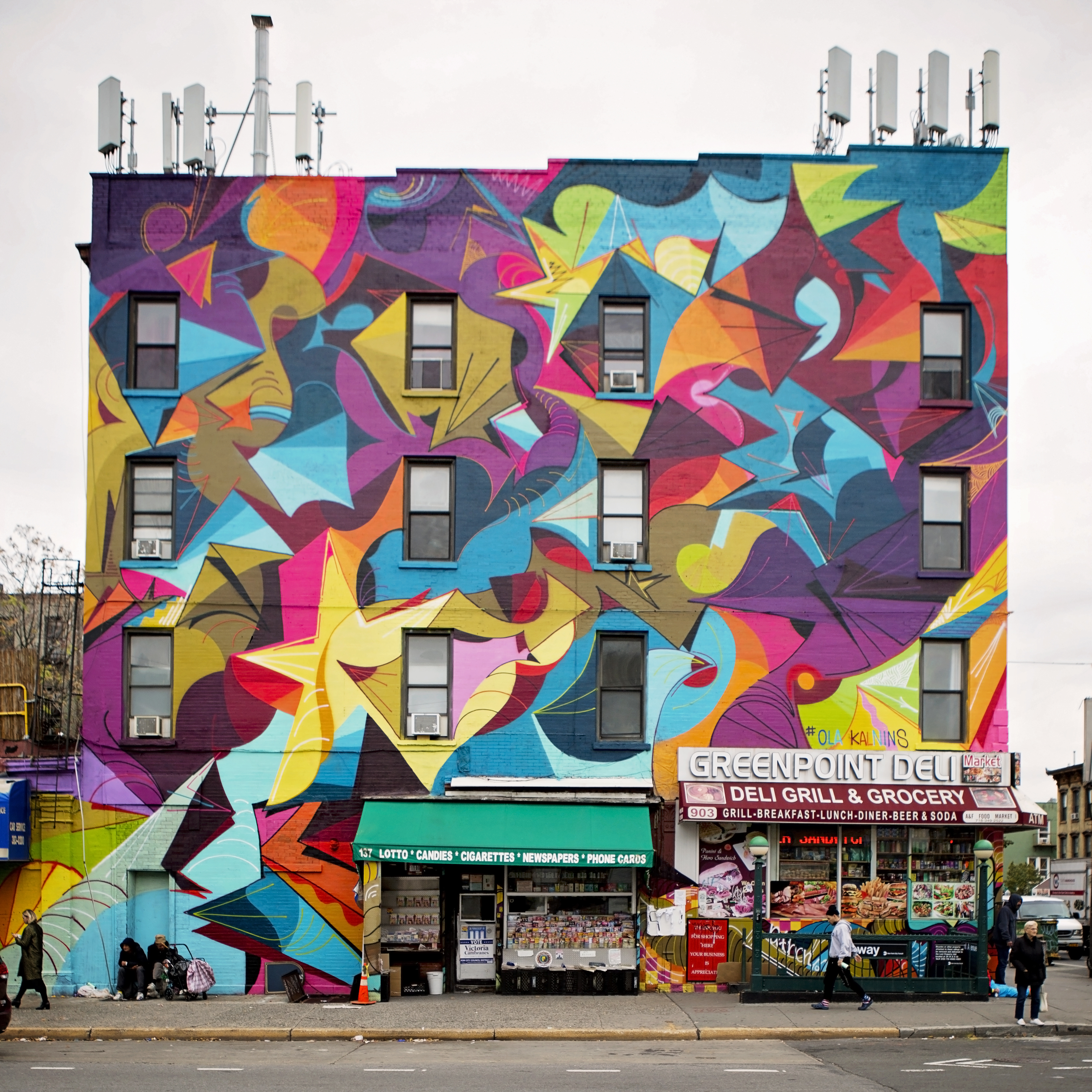This image captures a vibrant, artistic street scene featuring the colorful facade of a four-story apartment building. The building dominates the square, slightly portrait-oriented frame, showcasing an array of abstract and swirly designs in bright yellows, purples, blues, and other vivid colors, reminiscent of an artist's canvas. Each floor has four windows, some with air conditioners, making a total of 12 windows visible.

At street level, the image includes two shops under the colorful facade. The first is the Greenpoint Deli Grill and Grocery, easily identifiable by its white sign and red awning that advertises breakfast, lunch, dinner, beer, and soda. The adjacent shop, featuring a green awning, offers lotto tickets, candies, and cigarettes, with some fruit displays in front. Pedestrians can be seen in the scene, including a lady in black waiting to cross the road, adding a touch of everyday life to the vibrant urban setting.